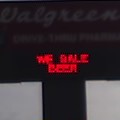The image is a very small and incredibly blurry picture, dominated primarily by black with some gray and faint text. The top portion of the image is black with a faint "Walgreens" sign. The middle section features a vertical black band flanked by gray squares. Below this, red digital-like text, reminiscent of an alarm clock's lettering, appears broken and hard to decipher. The red text seems to read "we sell beer," though the fragmentation makes it difficult to be certain. The image suggests a night-time setting, with the dark background and faint visibility contributing to the overall obscurity. Additional faint gray text seems to be present but is not readable due to the poor quality and small size of the image.